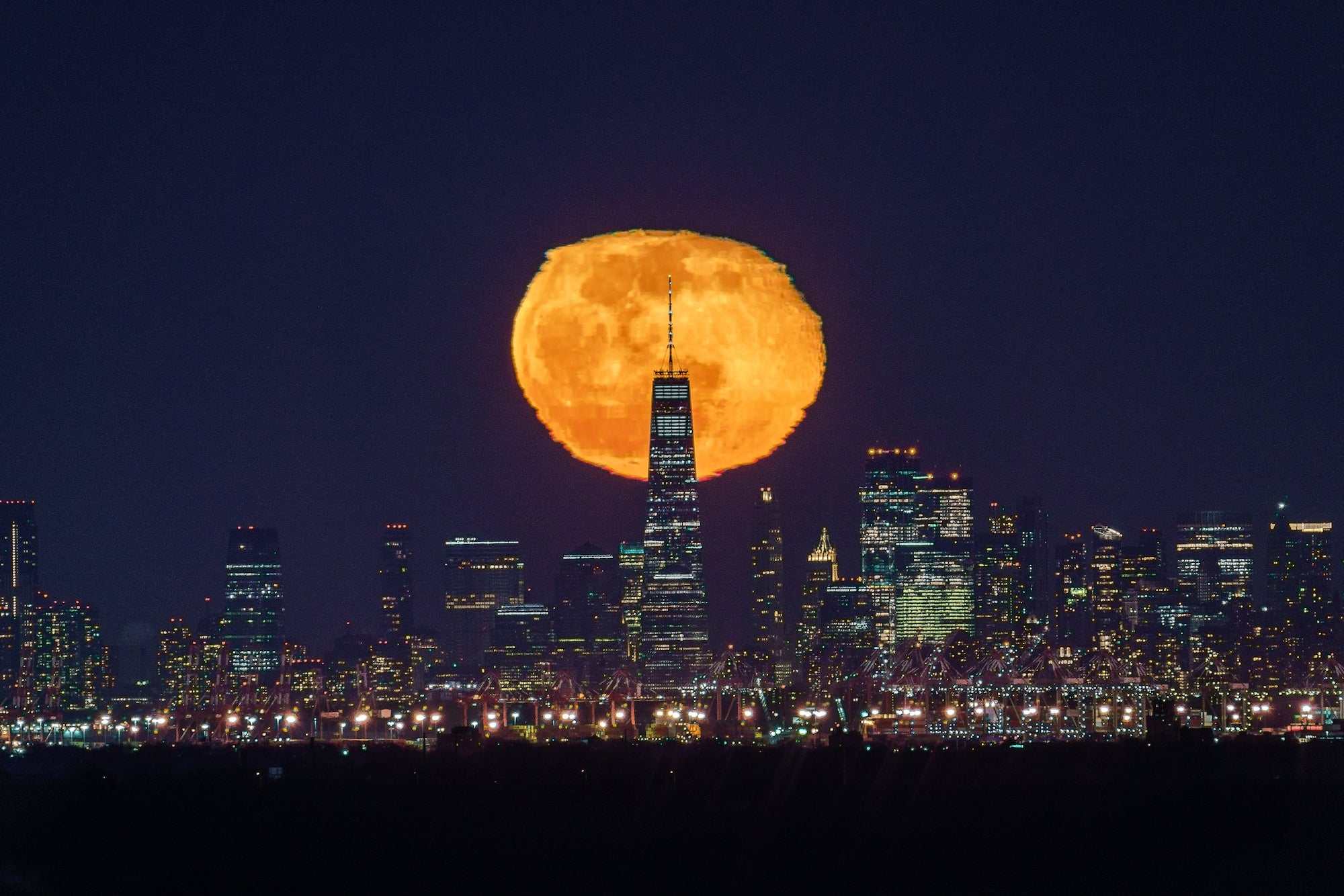This image showcases a nighttime cityscape dominated by towering skyscrapers adorned with colorful illuminated windows—yellow, blue, and greenish hues prominently visible. The tallest building in the center features a long point at its peak, while its upper sections are distinguished by blue windows, contrasting with the structure's overall black appearance. Stretching across the image, from left to right, a swath of black at the bottom suggests a shadowy foreground possibly dotted with small, indistinct trees and houses. The night sky above is a striking grayish-purple, intensifying to more purple towards the core where an unusual, distorted celestial body—perhaps a moon—is located. This object, resembling a fireball with orange and yellow tones, appears peculiarly pixelized and squished, disrupting its circular form. The peculiar nature of this 'moon' starkly contrasts with the silhouetted skyline below, which is also bathed in the deep darkness of the night, void of any stars due to light pollution.